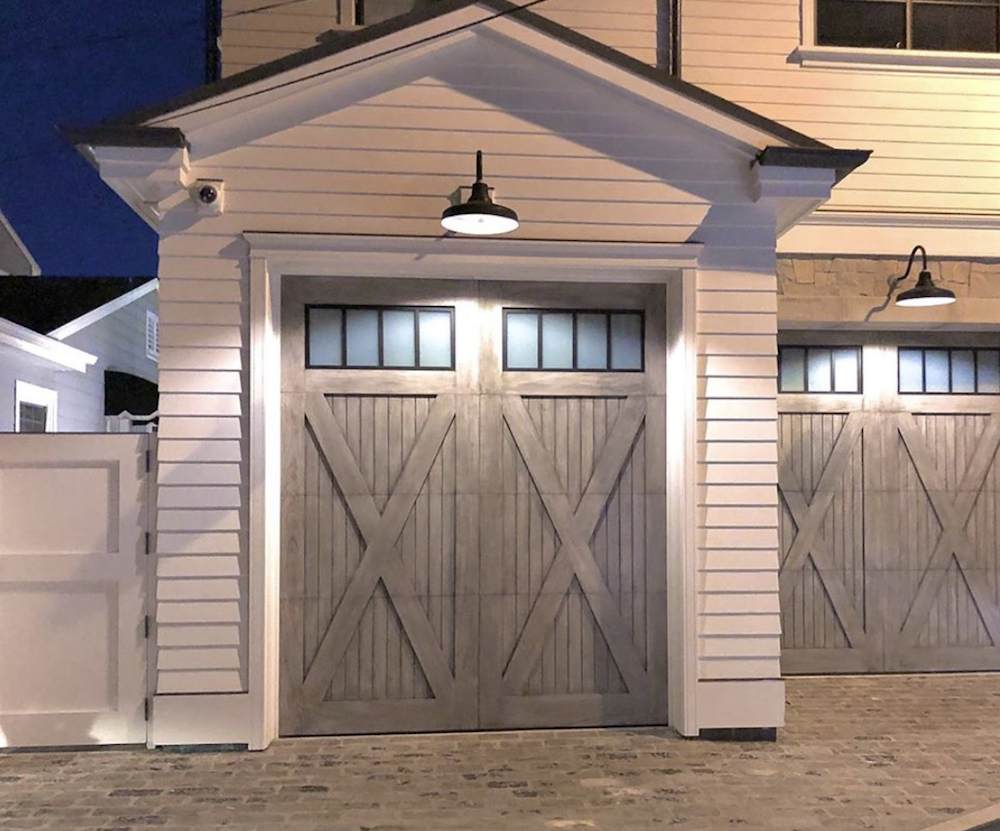The image depicts an outdoor nighttime scene featuring the side of a modern house. The focal point is a pair of barn-style garage doors, each with distinctive design features: four privacy-pane windows along the top and an "X" design made from wooden slats on the bottom. These doors are situated under a steep black-shingled roof. The house features light-colored siding, possibly white or light gray, accented by a warm, burnished gold light fixture. The lantern-like fixture sheds a bright, wide arc of light over the scene. On the left, a light-colored gate, possibly tan or cream, adjoins the garage and stands in contrast to a darker, neighboring house with a dark roof. The scene is framed by a deep blue night sky, enhancing the serene and inviting ambiance of the setting.